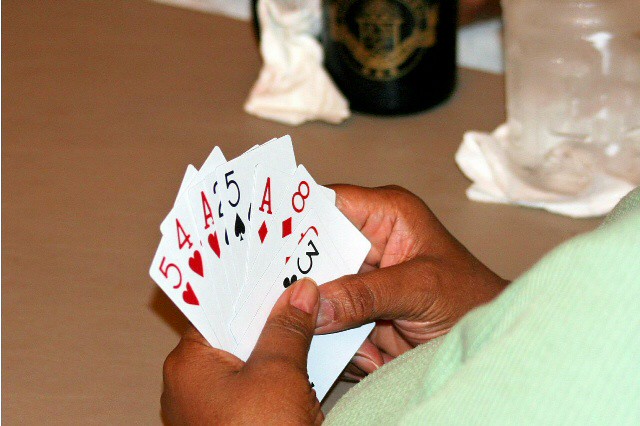A person is holding an array of playing cards in both hands, fanned out but slightly disheveled, as though needing a bit more adjustment to achieve a perfect spread. The cards, displayed from left to right, include the Five of Hearts, Four of Hearts, Ace of Hearts, Two of Spades, Five of Spades, Ace of Diamonds, Eight of Diamonds, Queen of Diamonds (partially obscured), and the Three of Clubs. The individual is positioned towards the right lower half of the image, facing left. In the background, a brown table is visible, bearing several items: a plastic drink bottle with a napkin underneath it, a black mug centrally placed, and another white cloth nearby. The setting suggests a casual, perhaps homey environment.